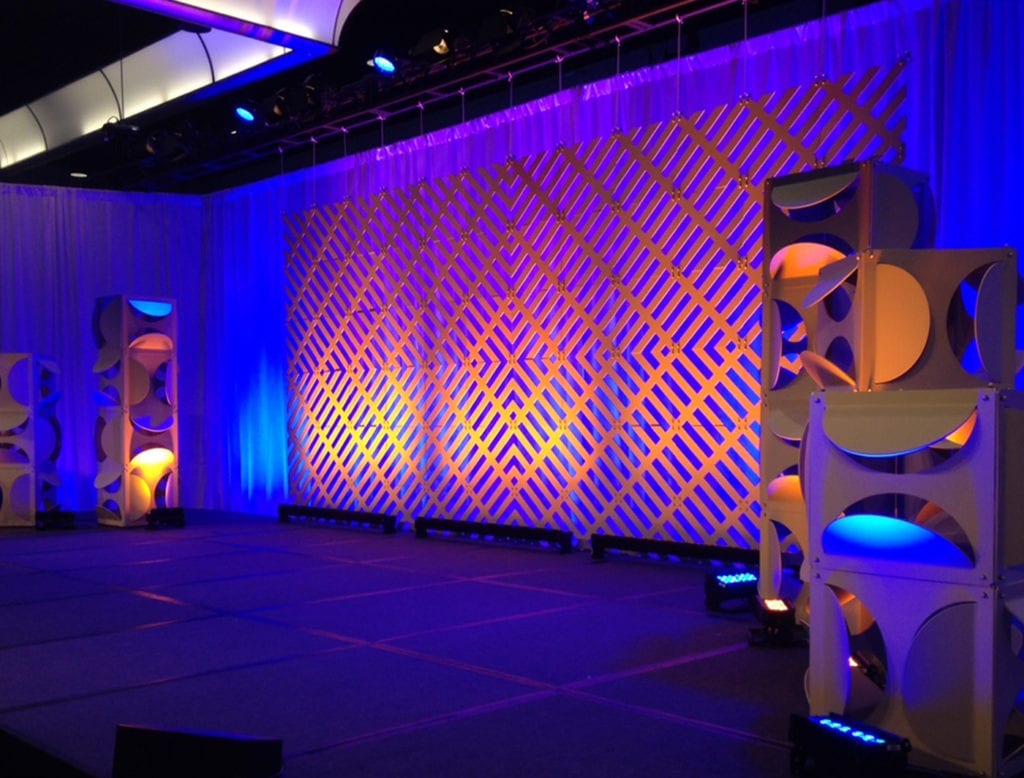The image depicts an empty stage adorned with a closed, neon blue curtain that spans the entire length and extends down the sides. The stage floor is a dark purple, accented with streaks of gold that reflect the lights. Above, there are mechanical catwalks and directed lighting, with circular blue lights shining down from the predominantly black ceiling. Geometric shapes and sculptures, possibly made of metal or wood, are arranged on either side of the stage. These modernistic sculptures exhibit open semicircles in four different places, with heights varying between six and eight feet. The background features a wide, gold-colored lattice structure with diamond shapes that increase in size towards the edges. Additional details include gold-colored speaker stands with yellow circular flaps, and in the upper left corner, a section of the roof with a white barrier and a light blue line underneath. Overall, the stage scene is bathed in a blend of neon blue, purple, gold, and bronze hues, creating a vivid and dynamic visual.